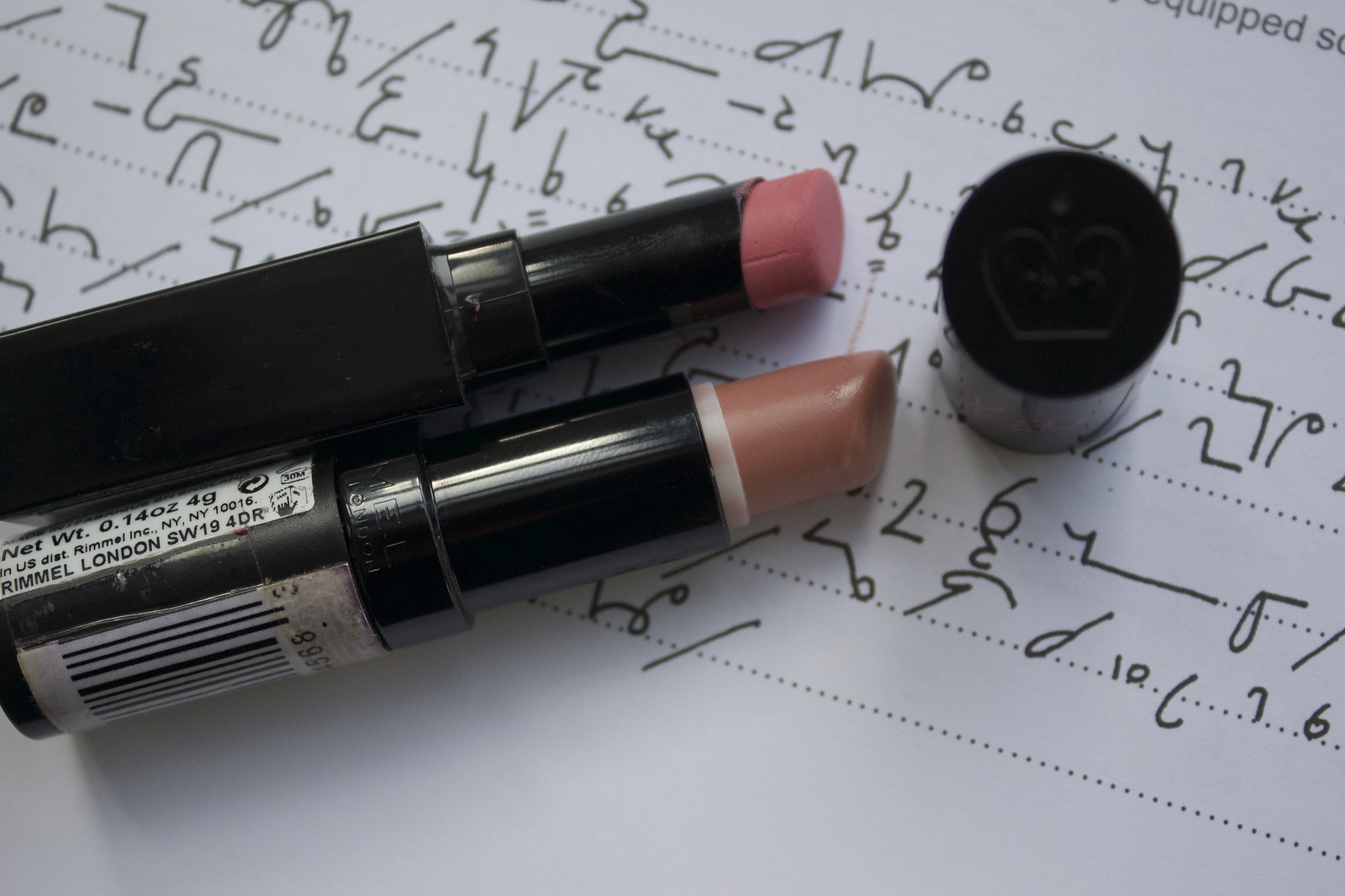The image features two lipsticks placed diagonally on a sheet of white paper with dotted lines and handwritten shorthand notes in black ink, featuring approximately seven lines of text. Both lipsticks are encased in solid black packaging. The top lipstick is a coral or dusty pink shade, while the bottom lipstick is a nude or beige color. The bottom lipstick still has a white and black barcode sticker with the code Rimmel London SW19 for DR on it. Additionally, the cap of one lipstick, which has a rounded top with an indented crown, is laying to the right of the nude lipstick. The paper beneath the lipsticks has small, hieroglyphic-like doodles, giving the scene a peculiar, almost mathematical feel.